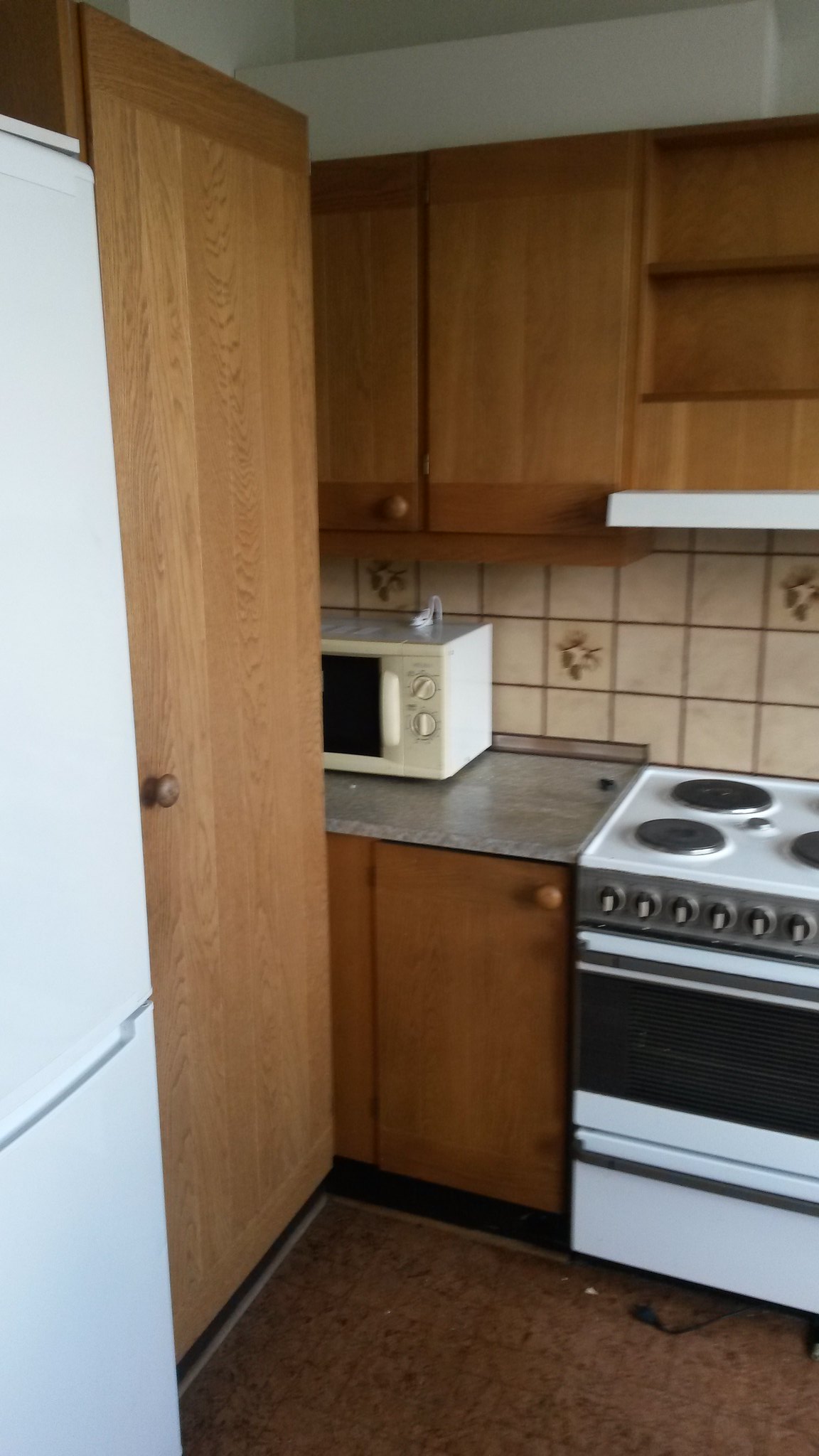This image depicts a small, narrow, and dated kitchen. The flooring is a beige-brown linoleum, appearing somewhat dirty with spots and an indistinguishable pattern. On the left side of the image, there is an impeccably clean white refrigerator adjacent to a tall cabinet with a wooden knob, resembling a door. A gray countertop runs beside the fridge, housing an old, yellowish-white microwave with two different knobs. This counter dead-ends next to a white oven featuring black and white knobs, with a plug hanging loose below it, suggesting it might be unplugged. Above the oven, there is a white built-in hood accompanied by a shallow wooden shelf. The backsplash behind the counter consists of tan tiles interspersed with a few designed tiles, completing the retro aesthetic.